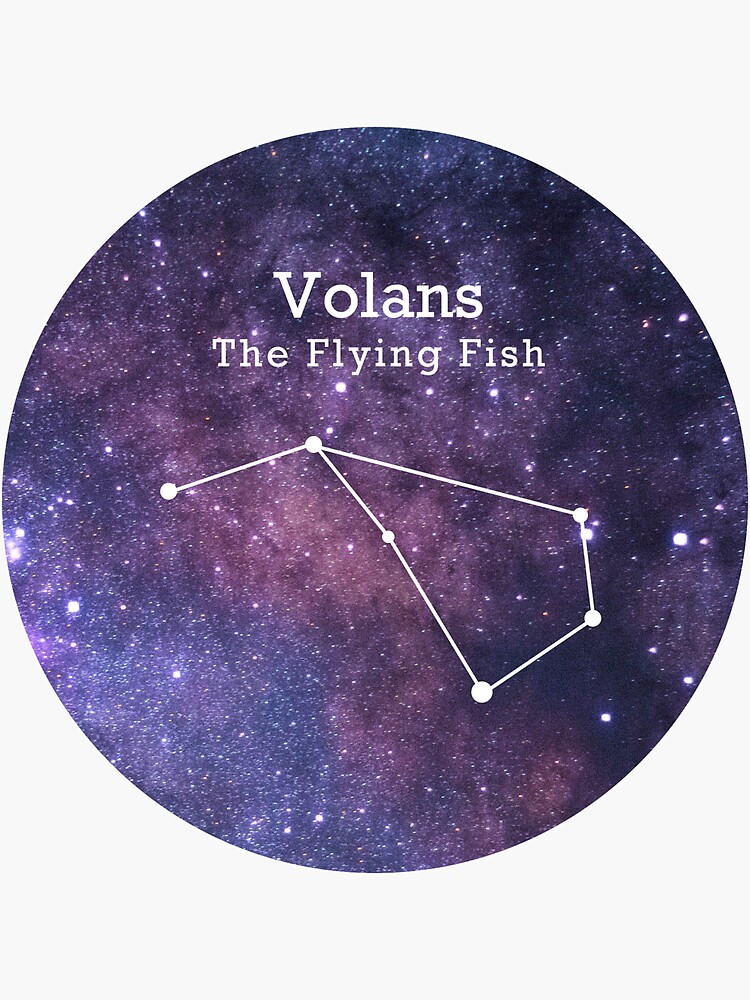The image is a detailed diagram of the Volans constellation, also known as "The Flying Fish." Set against a backdrop of dark blues, purples, and blacks, the circular image vividly depicts a region of space filled with variously sized white dots representing distant stars. The constellation itself is marked by large, white letters at the top of the image, spelling out "Volans," while beneath it, slightly smaller letters read "The Flying Fish." 

The constellation is illustrated with six connected stars, highlighted with white circles and interconnected by white lines. Starting from the middle left side of the image and extending diagonally upwards to the right, the stars form a shape that resembles an upside-down cup or a sideways kite. The mesmerizing cosmic background enhances the visibility of the constellation, making it stand out in stark contrast to the star-studded night sky.